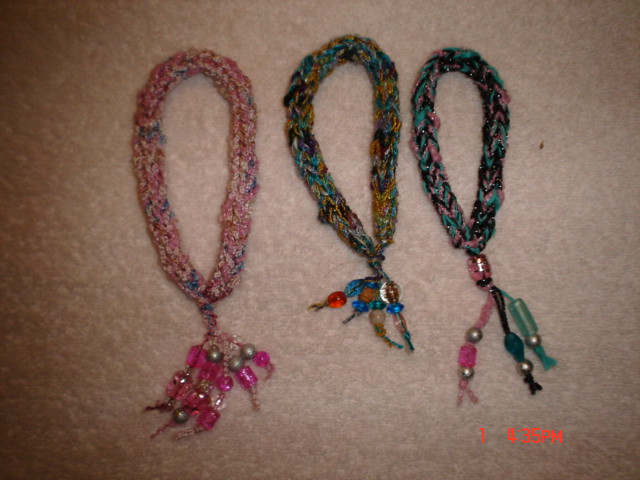This close-up photograph, though quite blurred and dark, displays three intricate, knitted fabric bracelets laid side-by-side on a cream-colored carpet. A time stamp in the lower right corner reads "4.35pm" alongside a red number "1". Each bracelet showcases detailed craftsmanship with loops and tassels, adorned with various beads. The first bracelet is predominantly pink, accented with white and blue specks, and has pink and gold beads hanging from it. The second bracelet features a mix of green, yellow, black, and grey yarn with blue, red, and clear beads. The third bracelet, highlighted with shades of blue, pink, and black, is decorated with pink, green, blue, and silver beads. These woven bracelets, likely handmade friendship bands, exhibit a charming and colorful array of inexpensive wrist art.